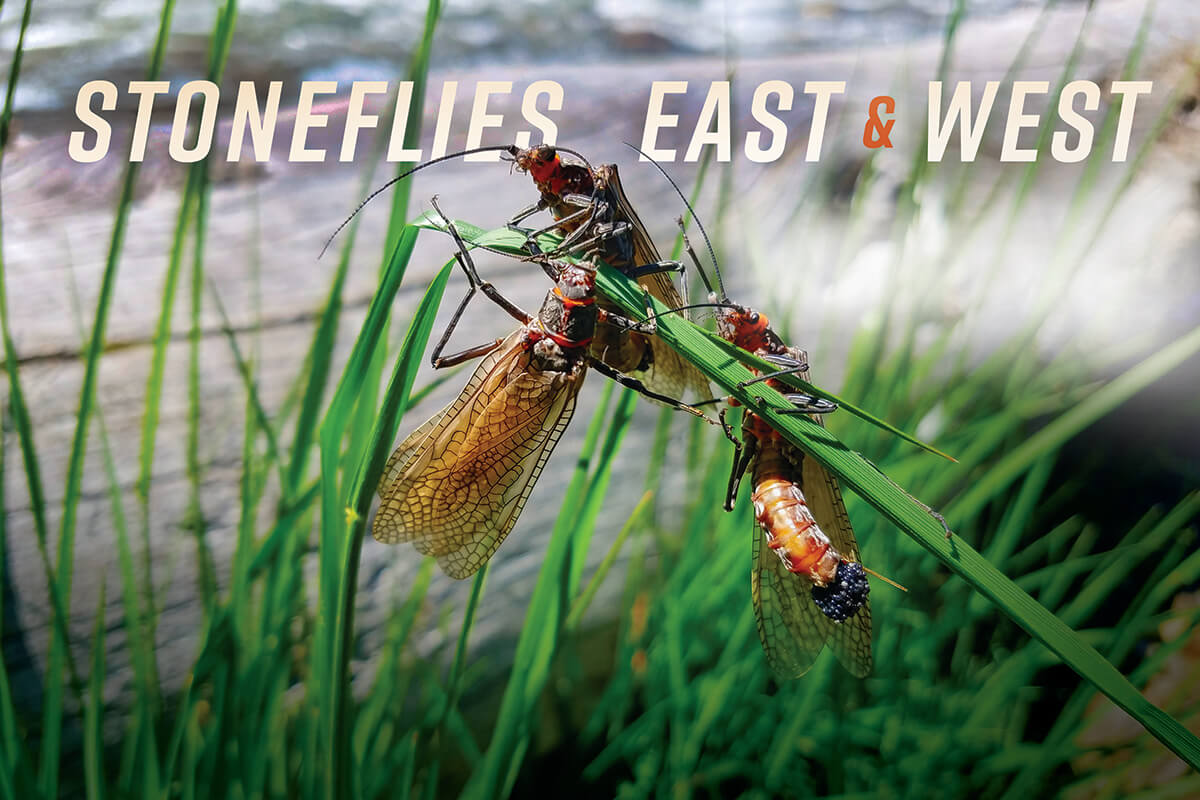The image features a vivid close-up of three or four stoneflies clinging to a blade of green grass. The photograph, a well-lit outdoor shot, has a shallow depth of field, sharply focusing on the insects while the background remains blurred. The stoneflies have reddish-orange bodies and conspicuous long, curved black antennae that adorn their heads. Their sizeable, slightly transparent beige wings display intricate patterns of segmented sections divided by black lines. The insects' large eyes add to their striking appearance. Some sections of the background include slightly focused tall grass, but most of it is out of focus, creating a muted gray backdrop. The top of the photograph features white text reading, "Stoneflies East and West."